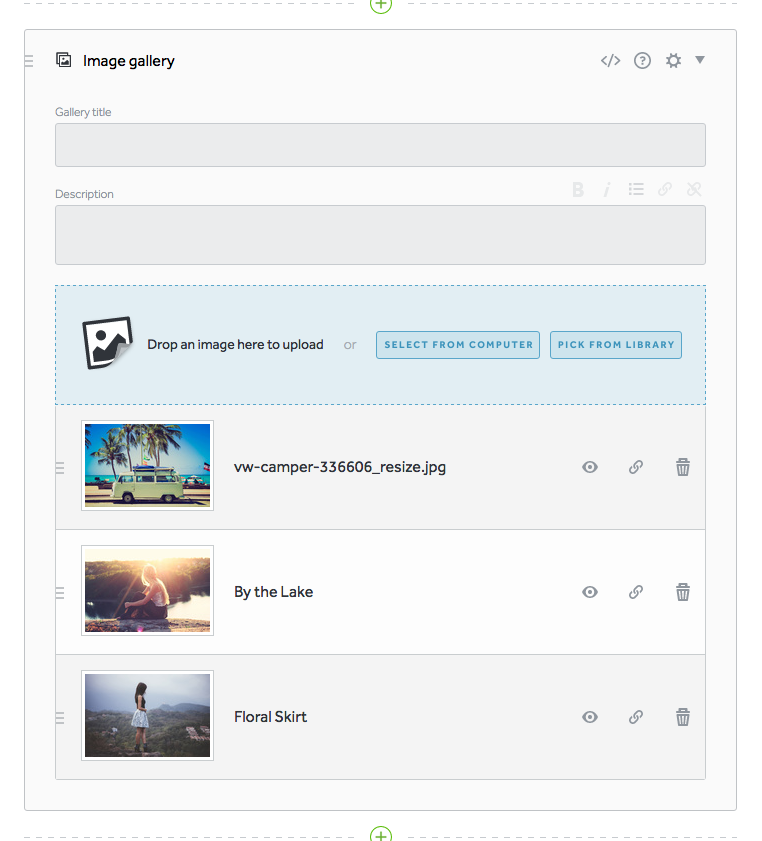The screenshot captures a vertically rectangular frame with a very light gray background, primarily focused on an image gallery interface. At the top left, the words "Image Gallery" are prominently displayed in bold black text. Below this title, there is a section labeled "Gallery Title," accompanied by a light gray field designed for entering the gallery's name. Following this, a section labeled "Description" appears, featuring a similarly shaded text field for additional details.

Further down, the interface presents a conspicuous light blue background area, which instructs users to "Drop an image here to upload," along with two buttons labeled "Select from Computer" and "Pick from Library."

Towards the bottom portion of the frame, three images are aligned vertically on the left side. To the right of each image, corresponding descriptions are provided. The first image is titled "VW-camper-336606_resize.jpeg," the second image is captioned "By the Lake," and the third is labeled "Floral Skirt."